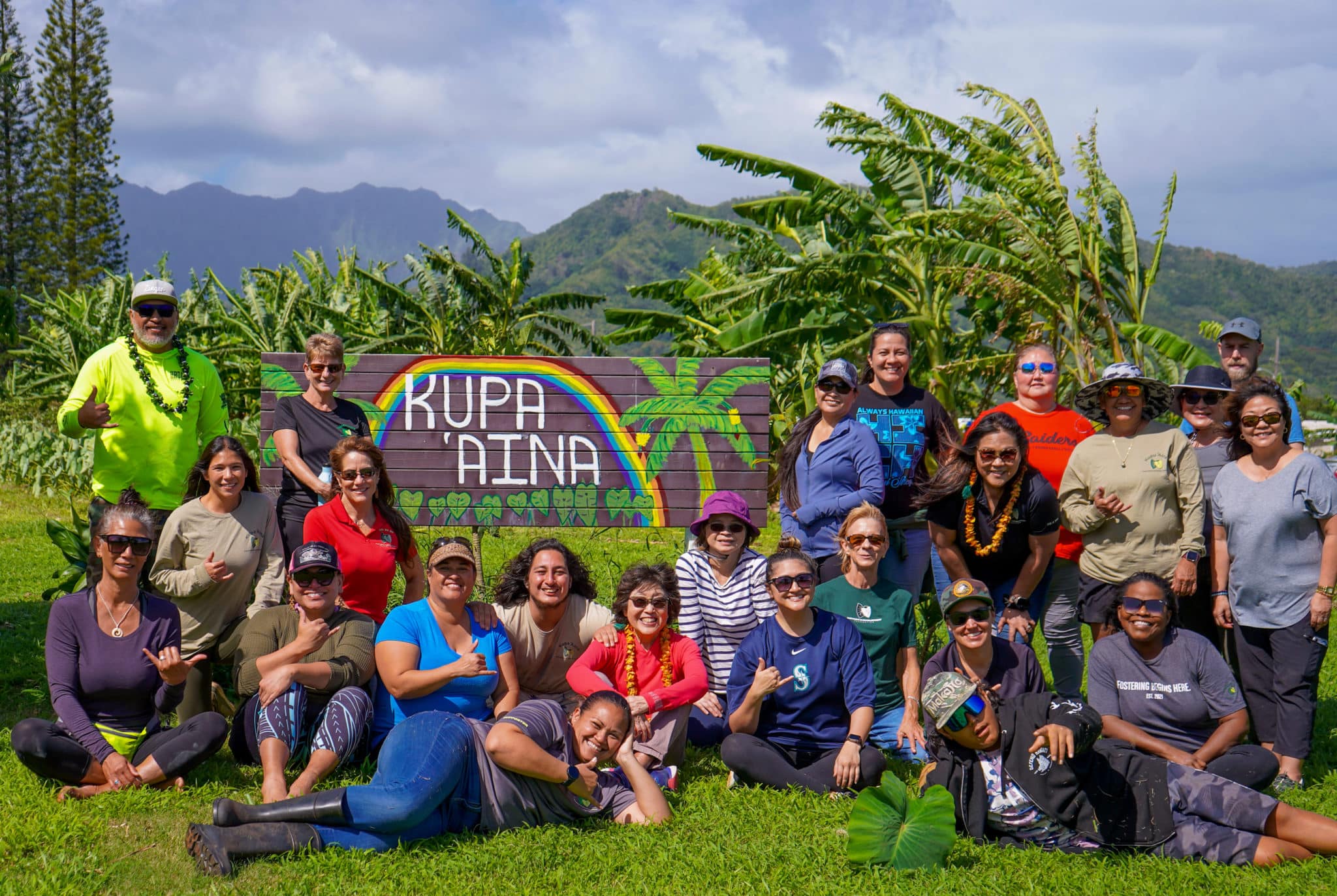In this vibrant group photo, a diverse assembly of people pose cheerfully in front of a large wooden sign that reads "Kupa'a Aina," adorned with a painted palm tree on the right and a rainbow arching over the white text. The sign is crafted from parallel brown wooden planks and is set against a lush, green backdrop. The group, consisting of individuals of various ages and genders, exhibits a variety of relaxed postures; some are standing, while others are sitting or laying on the short green grass.

A woman on the front left, distinct in her dark black boots, blue jeans, and purple shirt, lounges with a smile, her thumb resting on her chin and her head supported by her right hand. She wears a black watch on her left wrist. On the bottom right, a man reclines in camouflage shorts, his sunglasses reflecting blue and green hues, and a black sweater open in the middle. He also wears a camouflage hat.

The scenic background behind the group enhances the image, displaying a landscape of swaying palm trees, lush green mountains, and rolling hills. The sky above is filled with dark gray clouds, suggesting impending or recent rain. This serene yet dynamic setting, combined with the lively group, embodies a quintessential Hawaiian ambiance.